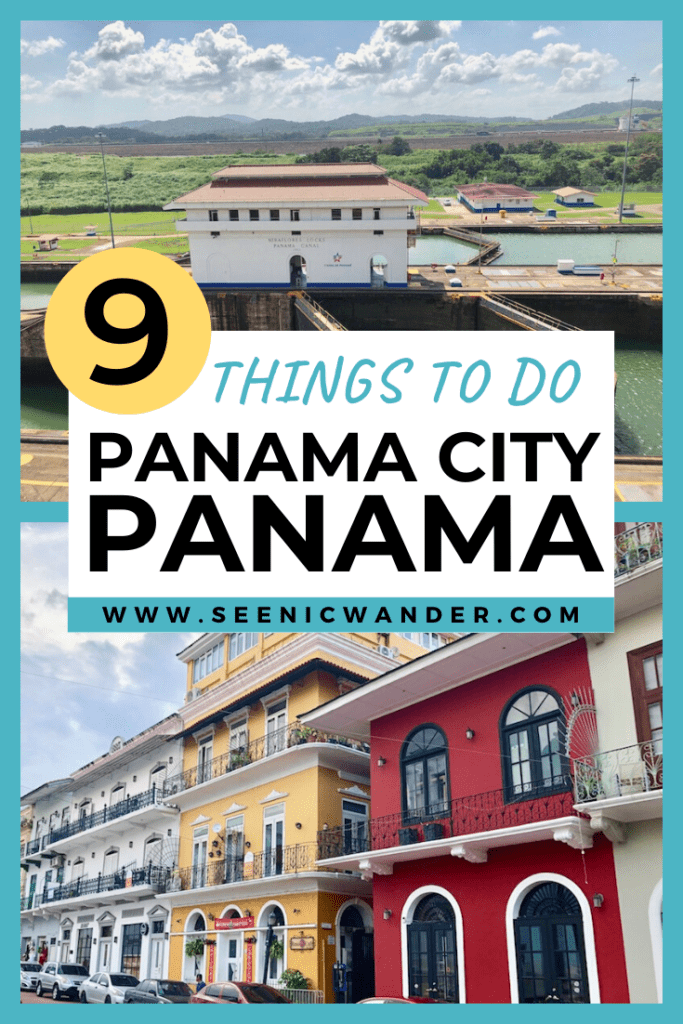### Discover the Charm of Panama City, Panama

**Top Image:**
A stunning white building with a distinctive brown roof stands gracefully over a serene body of water, reflecting its majesty. The structure, with its gray concrete foundation, offers a beautiful contrast to the vibrant blue sky overhead. In the background, lush green mountains dip into puffy white clouds, completing the picturesque scene.

**Middle Section:**
Nestled between the two captivating images, a white informational box draws your attention. In stylish teal and black font, it features a gold circle etched with the number nine. The heading in teal reads, "Things to Do," followed by "Panama City, Panama" boldly in black. Below, a teal and white section displays the website "www.cnikwander.com" in black.

**Bottom Image:**
A lively collage of colorful buildings evokes the atmospheric charm akin to French New Orleans. The architectural medley includes a pristine white structure accentuated with black railings, a regal gold-yellow building with matching black railings, and a striking red edifice featuring rounded black windows and gothic-style wrought iron details. Completing the ensemble, a pure white building with brown window frames and gray railings provides an elegant touch. Below the vibrant facades, various cars in silver, red, and black add a glimpse of everyday life in this vibrant, historic section of Panama City.

### Explore More at www.cnikwander.com